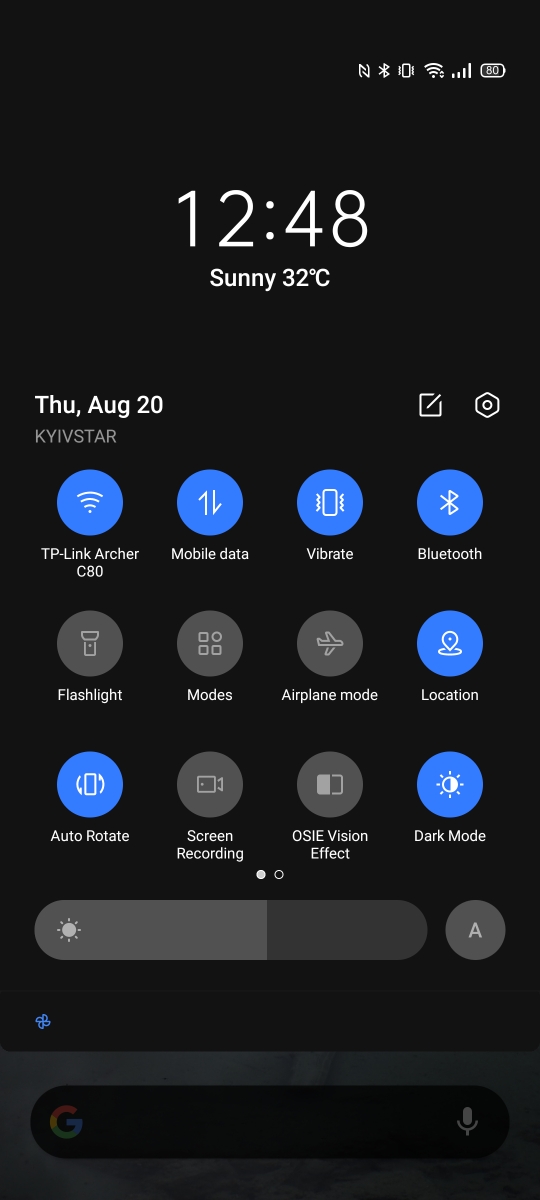**Detailed Caption for a Smartphone Home Screen Image under "Websites" Category:**

The image displays a smartphone home screen with specific settings and notifications visible. At the top of the screen, icons indicate that Bluetooth and Wi-Fi are enabled, the device is on vibrate mode, and the battery is nearly depleted. The current time is 12:48, though it doesn't specify AM or PM. However, given the indication of sunny weather and a temperature of 32 degrees Celsius, it is safe to assume it is 12:48 PM. 

Displayed prominently are the date and network provider information: Thursday, August 20th, connected to KYIV STAR. The home screen also shows various highlighted icons and settings: 

- **Wi-Fi** (connected to TP-Link Anchor)
- **Mobile Data**
- **Bluetooth**
- **Vibration**

These settings are highlighted in blue, denoting they are active. Other icons such as the flashlight, modes, airplane mode, vision effect, and screen recording are gray, indicating they are inactive. The location and dark mode settings are enabled, while auto-rotate is active. Additionally, the screen displays the current brightness level, and there is a settings button presumably offering deeper customization options for the device.

Overall, the image provides a detailed snapshot of the phone's home screen status and active settings.